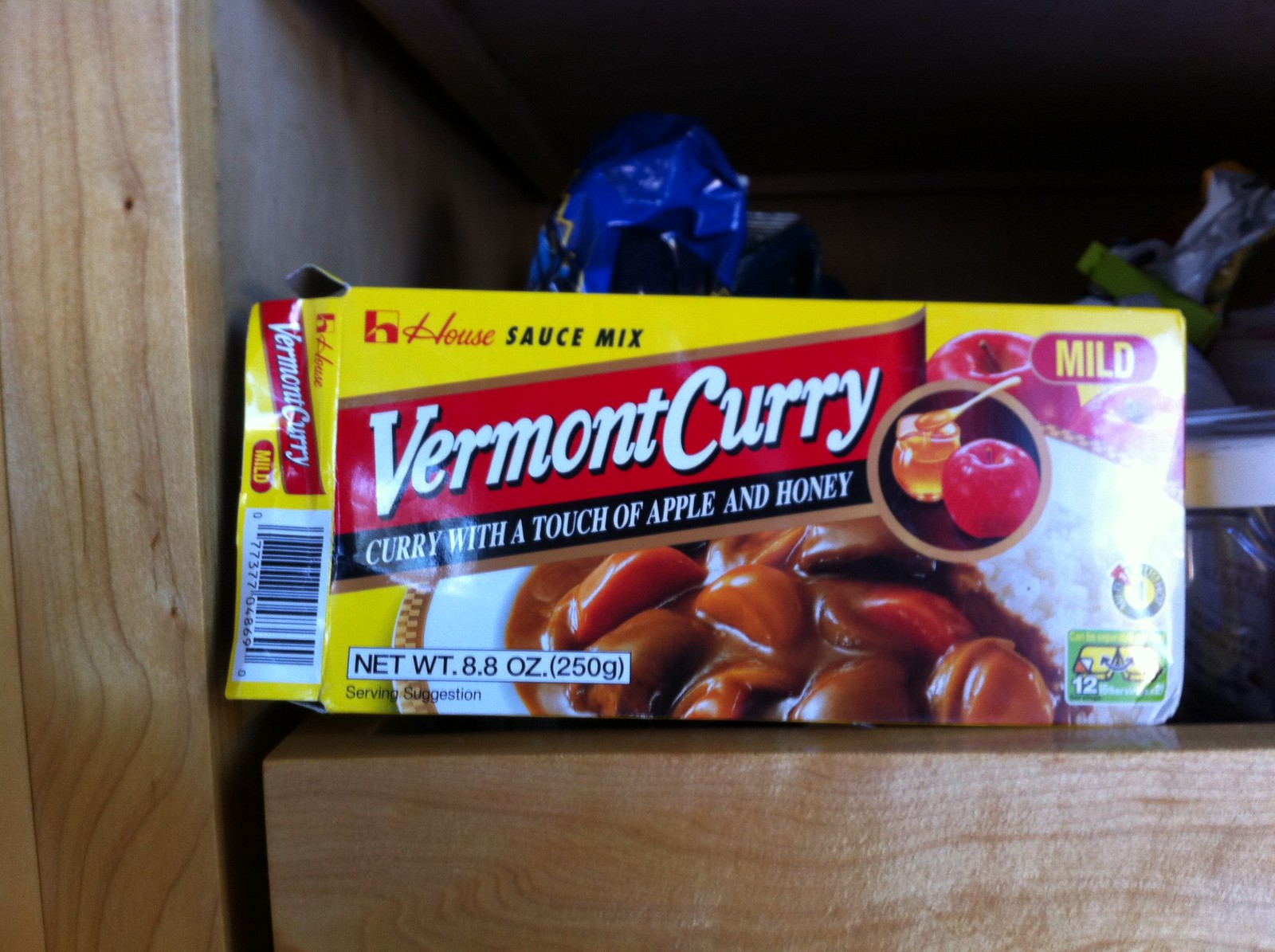This image is a close-up of a rectangular yellow box of Vermont Curry with a touch of apple and honey, sitting on a light brown wooden shelf, likely in a pantry. The box prominently features a red banner with the text "Vermont Curry" in white, and just below, within a black border, it reads "curry with a touch of apple and honey." The top left corner displays the logo "House" and the description "sauce mix." The top right corner indicates the flavor as "mild." The front of the box also includes a circular image showing a jar of honey with a spoon, placed next to an apple. Additionally, there is an image of gravy spread over rice, suggesting a serving idea. The bottom left corner details the net weight of the product as 8.8 ounces (250 grams), and the lower right section features two diagrams which are somewhat obscured by a light glare. Behind and around the box, various bagged pantry items are visible, including blue-colored and yellow-clipped bags, further suggesting the setting of a kitchen pantry.